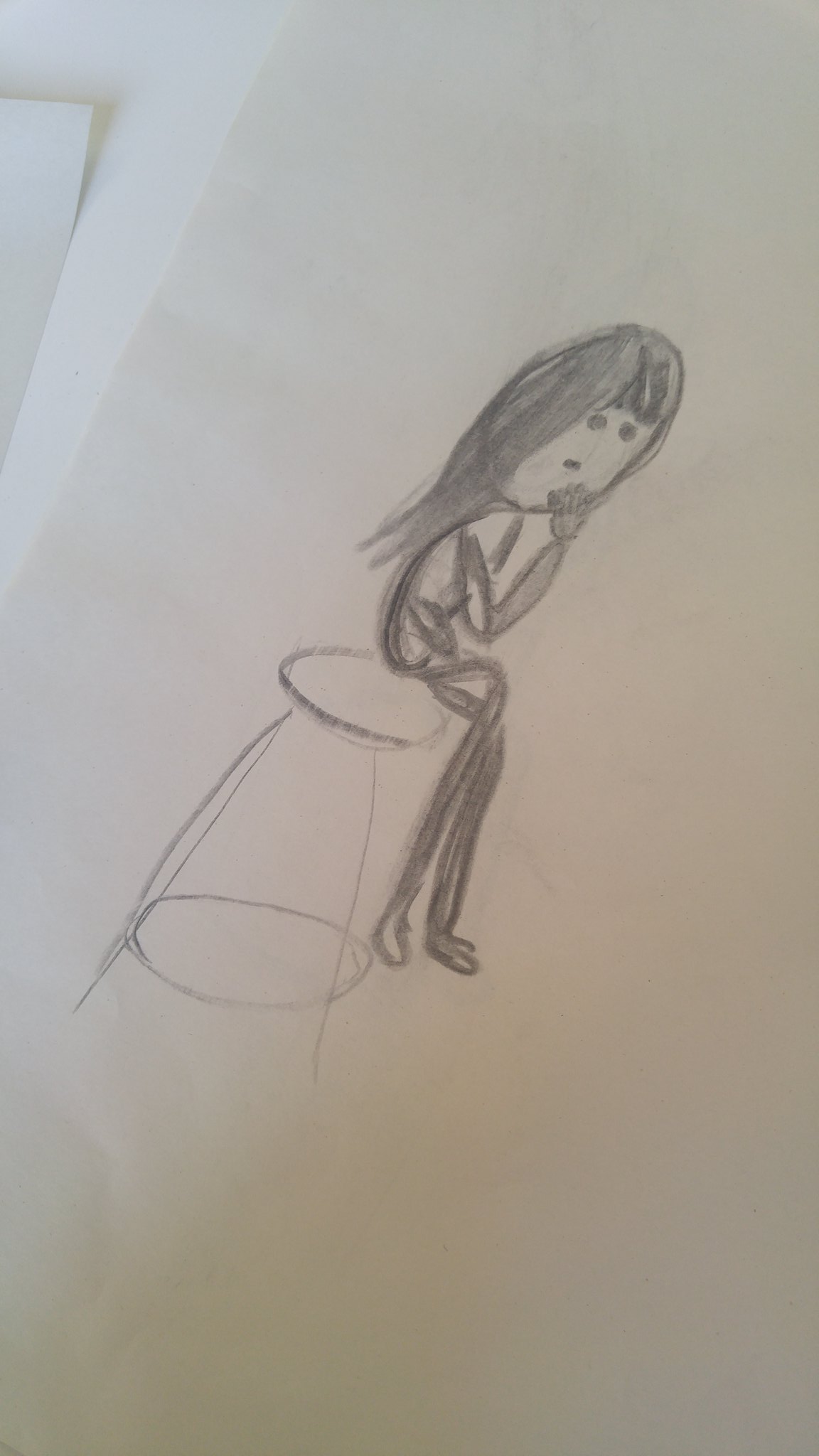This image showcases a simple pencil sketch of a girl drawn on a plain white piece of paper, which is resting on a similarly white surface. The girl has long hair that reaches the middle of her back and straight bangs framing her forehead. Her facial features are minimalistic, consisting of two small dots for eyes and a very tiny line for a mouth, giving her a somewhat pensive expression. She is seated on a round-seated stool with a larger circular base, appearing to have crossed her legs and bent one arm at the elbow, with her hand thoughtfully brought up to her chin. The sketch captures the girl in a moment of contemplation with a basic stick-figure style, using shades of gray characteristic of pencil or possibly charcoal. Additionally, a part of another piece of paper can be seen in the upper left corner, confirming that the sketch occupies the central area of the paper and is oriented in portrait mode.